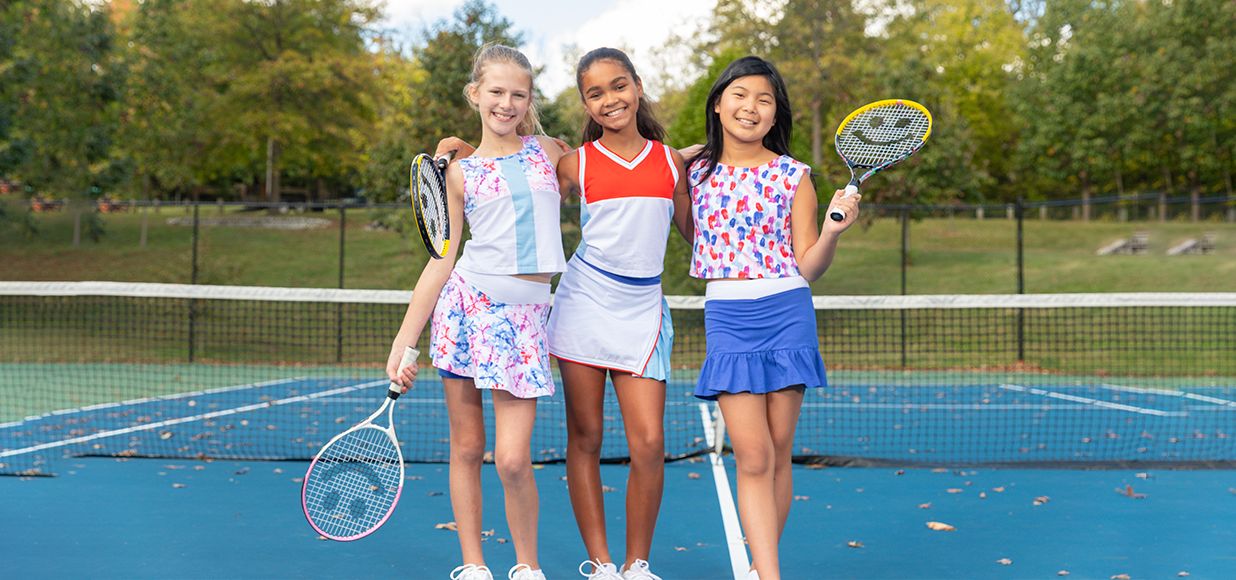The image captures a vibrant and cheerful scene on an outdoor tennis court where three young girls, roughly aged 10 to 12, are posing with their arms around each other. They are centered in the image and stand in front of a black tennis net with a white band at the top. Each girl holds a small, mesh tennis racket featuring a distinctive black smiley face. 

From left to right, the girl on the far left is white with blonde hair, wearing a white outfit adorned with floral designs—specifically a floral skirt and a white top with a light blue stripe down the middle and floral patterns on the shoulders. The girl in the middle, with a darker complexion and dark hair, wears a short-sleeved red and white outfit, paired with a white skirt that has a blue area design on the side. The girl on the right, who appears to be Asian and has dark hair, dons a sleeveless floral print shirt and a blue skirt accented with a white band.

The tennis court itself is blue and speckled with fallen leaves. Behind the girls, a metal fence encloses the court, beyond which lies a grassy hill interspersed with trees. The backdrop is a lush tree line under a sky that peeks through the foliage, adding to the serene and picturesque setting.